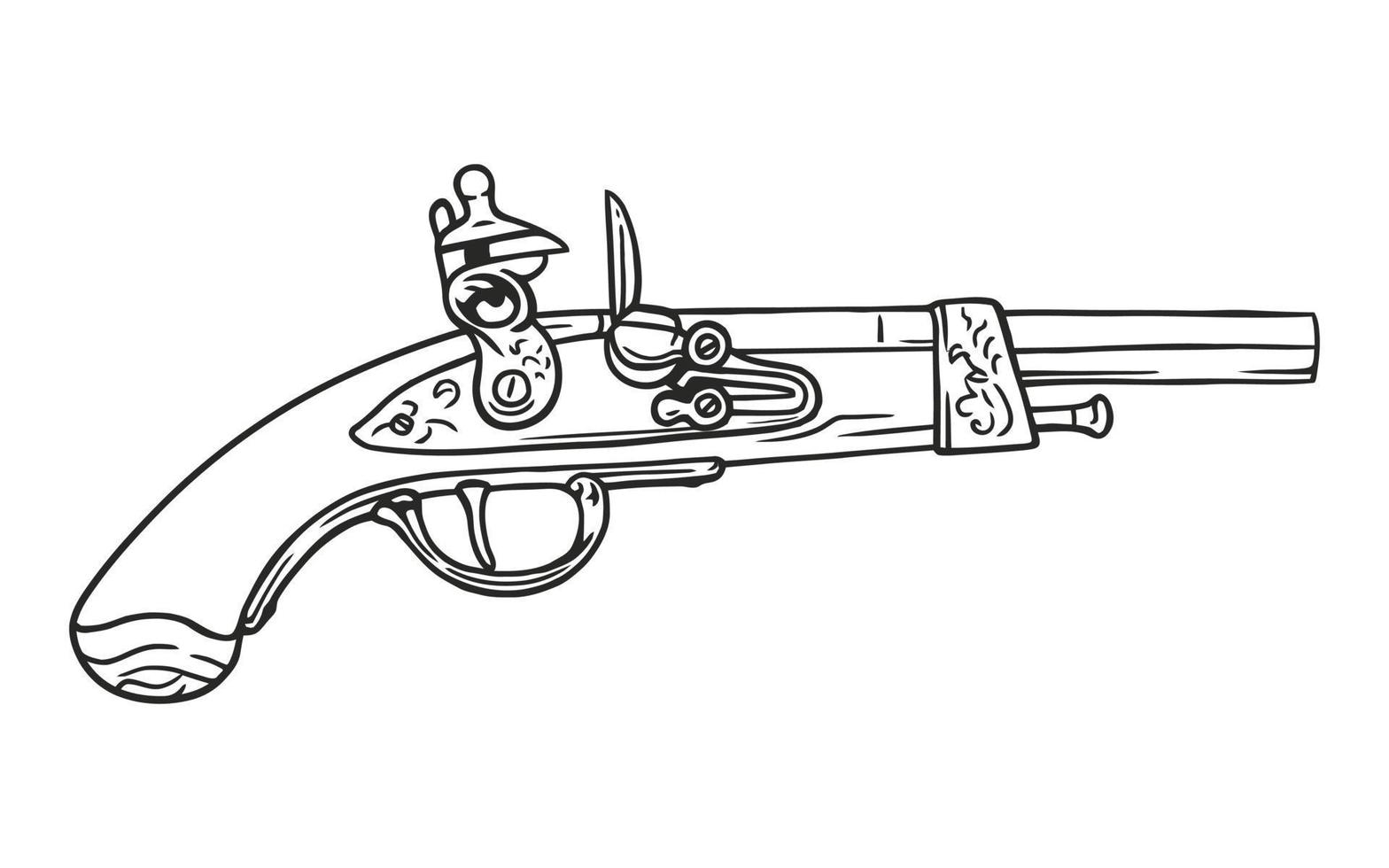This is a detailed line drawing of an antique flintlock pistol, illustrated in black ink on a white background. The sketch meticulously depicts the right side of the pistol, showcasing various intricate components such as the trigger, hammer, and pan. The barrel and muzzle are clearly outlined, along with the ramrod protruding from beneath the barrel. Sparse details attempt to represent the wood grain of the handle, highlighting its minimalistic engraving. Visible attachment points and screws meticulously connect the parts to the stock of the gun. Despite being a handheld pistol rather than a rifle, the illustration may cause some confusion due to its detailed depiction and elongated barrel. The overall design is simple yet precise, capturing the essence of the antique firearm.